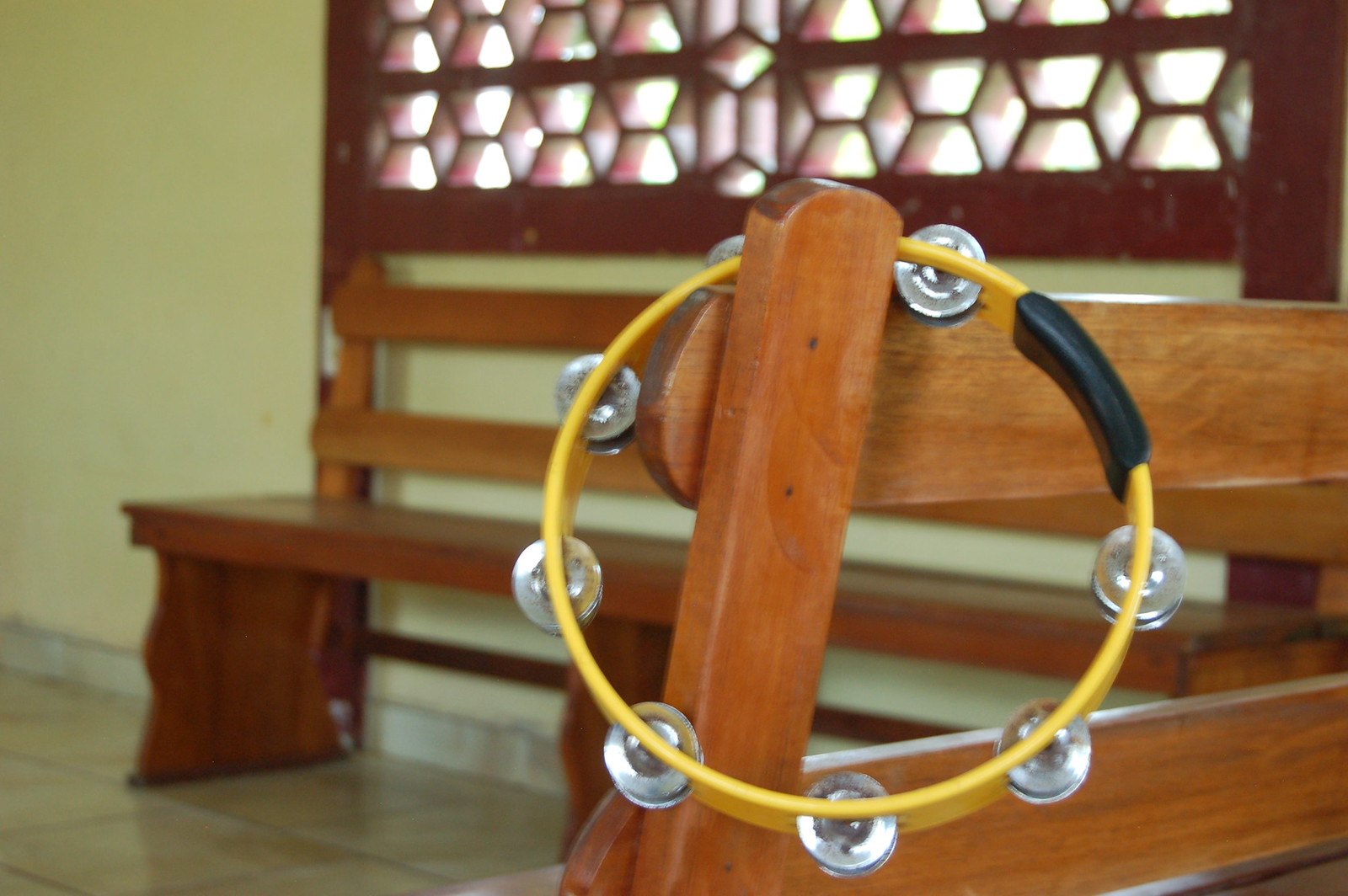The photograph captures an indoor scene featuring a polished wooden bench with a shiny lacquer finish, positioned prominently against a yellow wall. In the background, another wooden bench stretches along the wall, forming an L-shape seating area. Above this seating area, there is a decorative arched section or possibly a window adorned with pink and white stained glass in a diamond pattern, allowing light to filter through. The floor is composed of ceramic tiles with a clean, shiny appearance. Attached to the backrest of the foreground bench is a bright yellow tambourine with a small black foam handle. The tambourine is detailed with approximately eight to nine silver jingles that glint in the light.